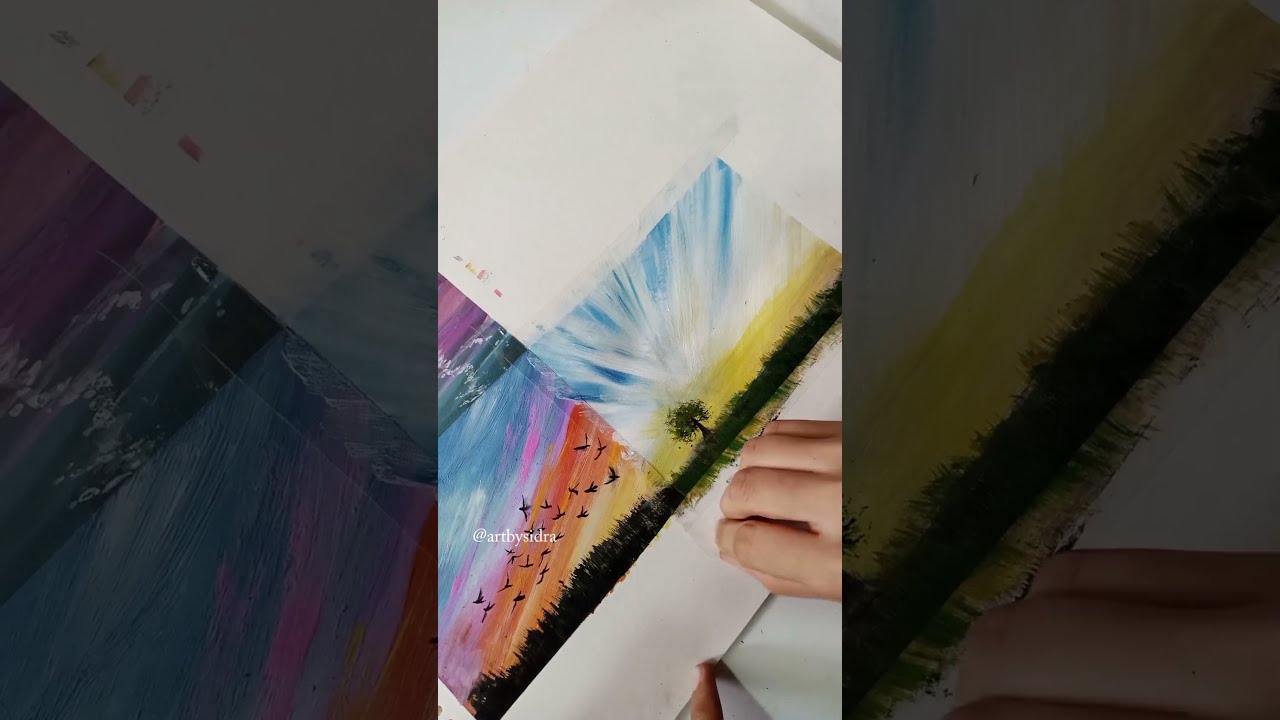This horizontally rectangular image features a central vertical strip depicting hand-painted artwork on a sheet of paper. A person's left hand is holding the artwork steady while their right hand points to specific details. The artwork portrays a vivid scene with an orange and blue sky, a green tree, grass, and a flock of black birds overhead. Surrounding the central strip, on the left side, there is a close-up of the sky, and on the right side, a close-up of the grass, both faded and darkened, serving as a background effect. Also included are parts of other paintings: a gold mountain range with a single black tree under a blue and white sky, and a partially visible section of another image with purple and green. The text "art by Sidra" appears at the bottom in white. The overall style is a photographic realism of hand-painted illustrations.